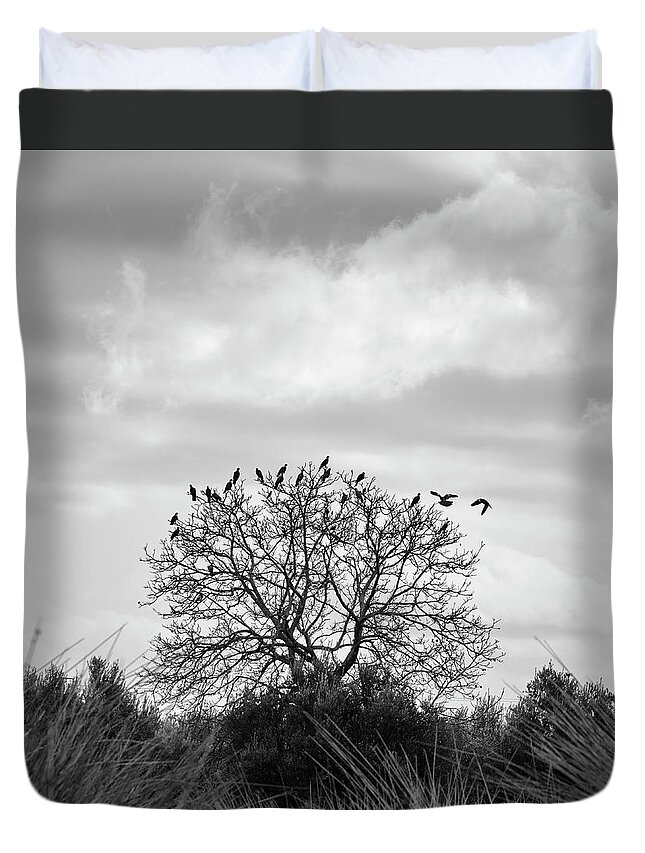This product photo captures a digitally altered graphic on a duvet cover, styled in a stark black and white color scheme. The centerpiece of the design is a bare tree with many branches, devoid of leaves, suggesting a winter setting. Perched along the top branches of the tree are numerous birds, some appearing to have just landed. The scene is framed by tall, dark grasses at the bottom of the comforter, with a backdrop of gray skies filled with clouds. The duvet cover features a thick black border at the top, adding a strong contrast to the monochromatic design. Two white pillows peek out from behind the duvet, providing a subtle touch of brightness to the otherwise Gothic ambiance. The entire image evokes a somber, Edgar Allan Poe-like aesthetic.